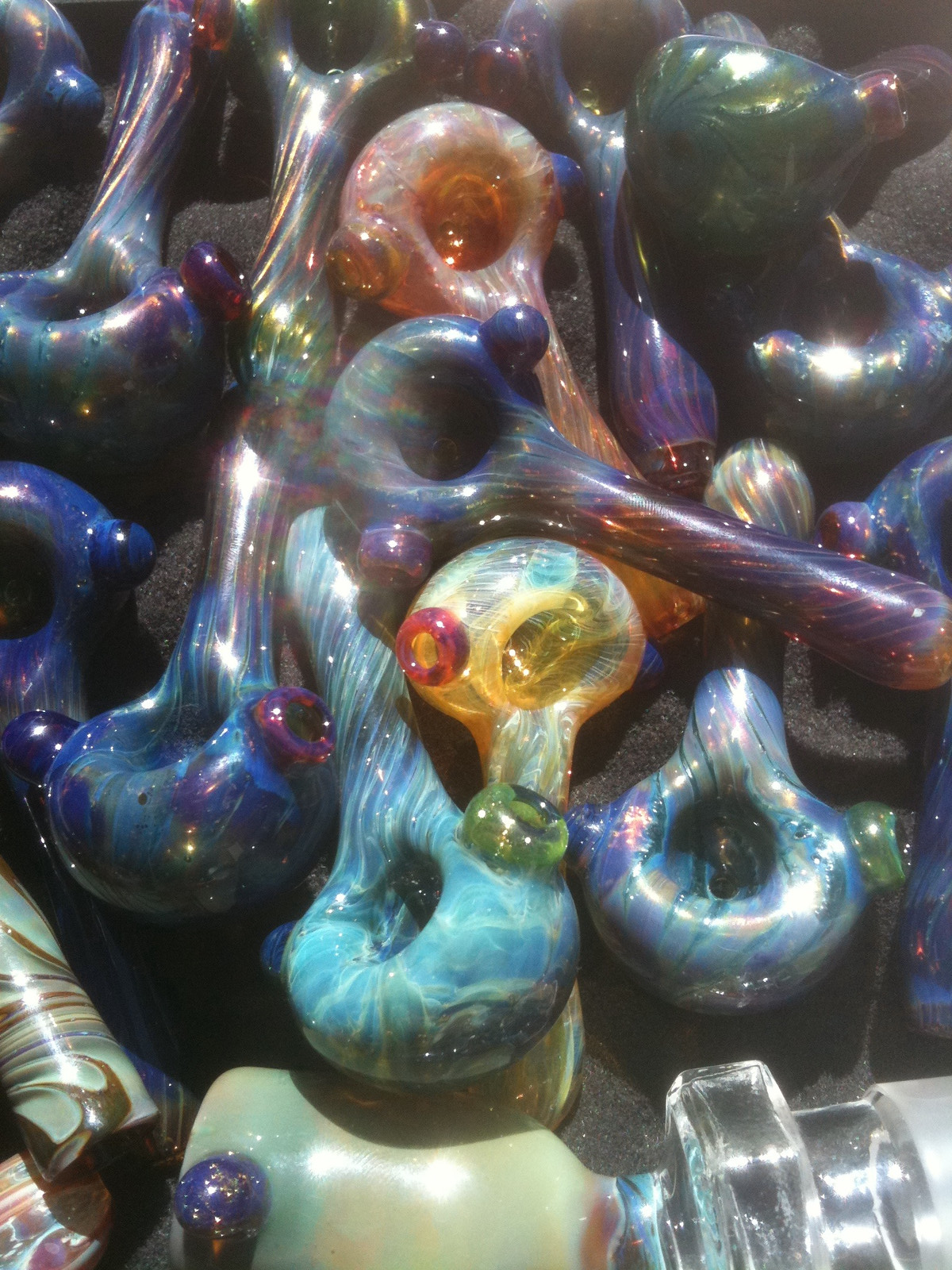This close-up photograph showcases a collection of approximately fifteen hand-blown glass smoking pipes. Each pipe features a bulbous bowl where tobacco or marijuana can be placed, and an elongated body. The pipes' unique and eccentric designs are characterized by a mesmerizing, swirled pattern in a dazzling array of colors, including blue, purple, red, yellow, teal, and orange. Many pipes exhibit a tie-dye effect, seamlessly blending multiple hues. The glass is likely translucent, giving the pieces a delicate, almost ethereal quality, enhanced by occasional sparkly accents. Scattered across a gray foam background, these intricate pipes are stacked upon each other, making the surface beneath barely visible. In addition to the uniform bowl and body design, several pipes feature small decorative knobs on the edges of the bowl area. Amid the abundance of pipes, one item stands out at the bottom of the image—an object resembling a small vase with a glass top, possibly another type of smoking device. The setting suggests a display, perhaps in a shop specializing in smoking paraphernalia.